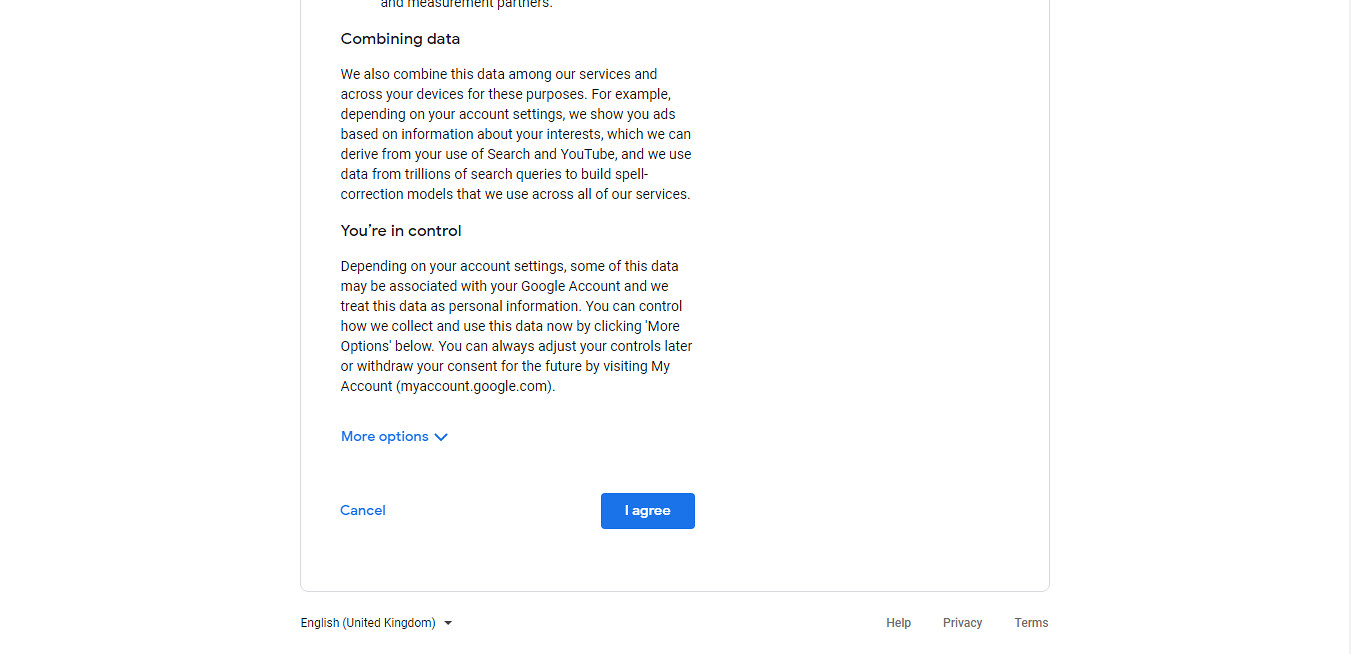The image features a white background with a document that has predominantly black text and some blue elements. The top section of the document is partially legible, with the text starting with "parties" and followed by "combining data." The document discusses how data is combined and utilized across various services and devices, highlighting personalized ad delivery based on user interests, derived from interactions with services such as YouTube and search engines. It mentions the use of data from trillions of search queries to improve spell correction models across all their services.

The document emphasizes user control over data collection and usage, noting that users can manage their data settings through their Google account. It assures users that they have the ability to adjust these settings, withdraw consent, and control their data by visiting myaccount.google.com.

Below the main text, there are two interactive elements in blue: "More options" with a clickable upside-down V, and "Cancel." There is also a prominent blue box with the text "I agree" in white, for users to consent to the terms. Outside the main outline of this textual content, there is additional text indicating the language setting as "English, United Kingdom," and links to "Help," "Privacy," and "Terms" on the far right side.